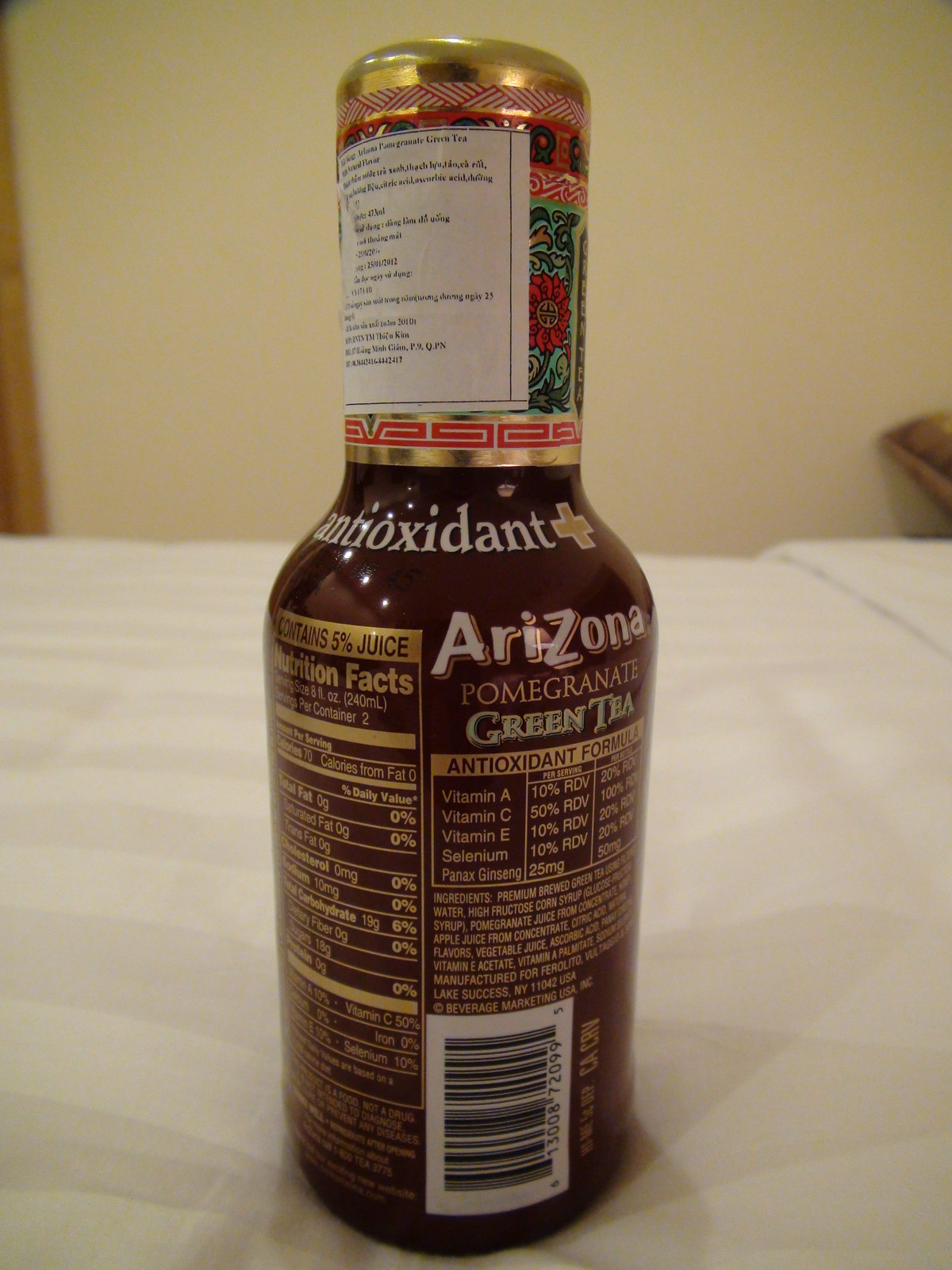The image captures an unopened bottle of Arizona Pomegranate Green Tea positioned on what appears to be a bedspread in a bedroom. The bottle features a distinctive green label with floral designs at the top right corner. The neck of the bottle, which is narrow for about two inches before widening, displays the word "antioxidant" followed by a tan plus symbol with a white border. The bottle's color is a dark reddish-brown, adorned with gold lettering. Below the floral design, the bottle proudly showcases the Arizona brand name with "A" and "Z" in uppercase and the remaining letters in lowercase. "Pomegranate" is prominently displayed in uppercase block letters, followed by "Green Tea" in light green letters with a shaded border. The side of the bottle reveals the nutritional facts and ingredients, with the barcode positioned towards the bottom, outlined in white. At the top of the bottle by the cap, there is a white label affixed, albeit the text on it is unclear. The image also includes a glimpse of a white square, possibly a piece of paper, and a waffle in the background.